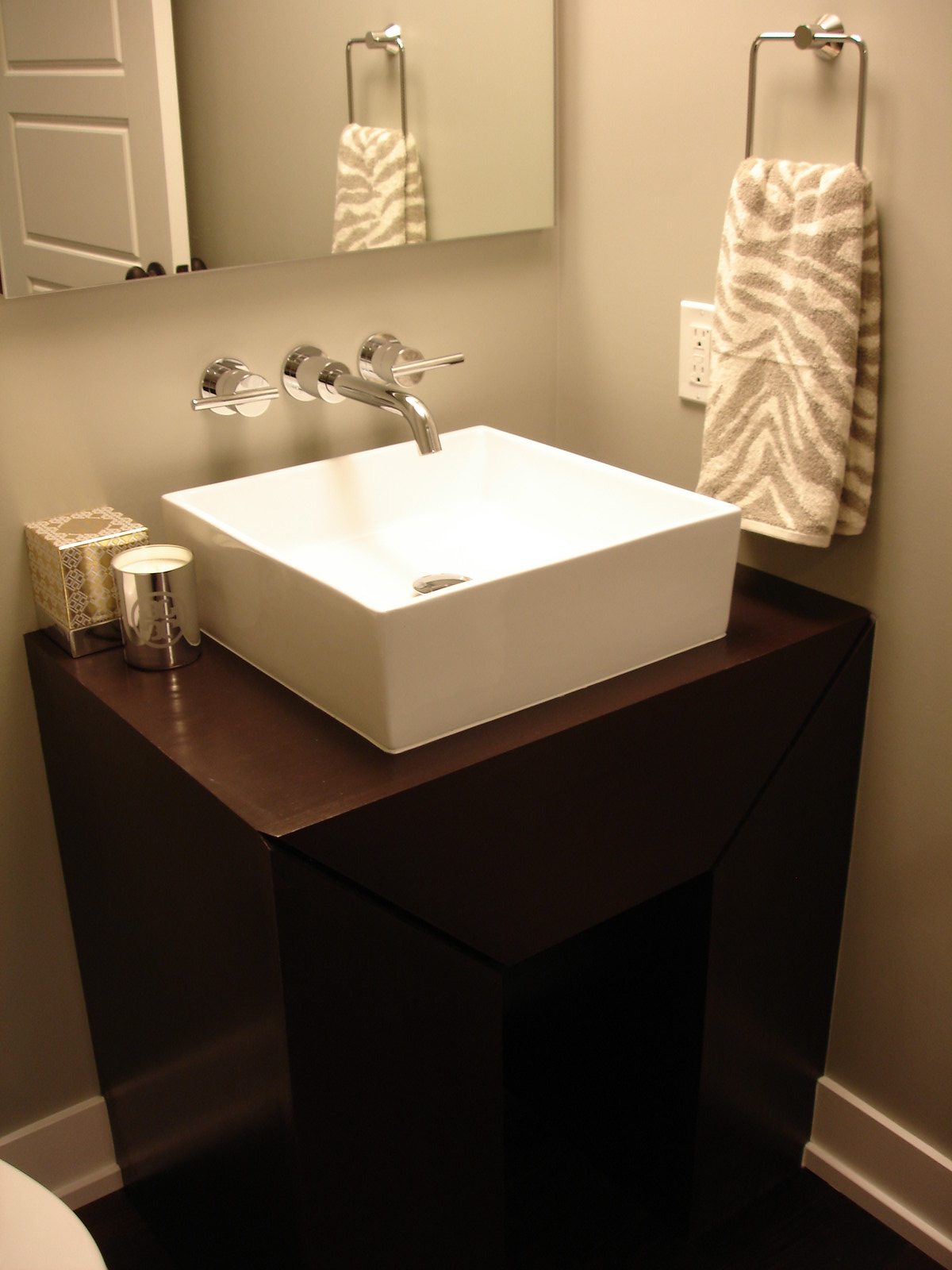This image depicts a small bathroom with grayish-colored walls and a white outlet area. A silver towel holder is mounted on the wall, displaying a zebra print towel in white and gray hues. A square-shaped mirror hangs on the wall, reflecting a white door, the towel, and the towel holder. Below the mirror, there is a vanity that features a wall-mounted hot and cold water faucet set above a deep, square-shaped sink placed atop the counter. Adjacent to the sink, there is a silver tissue box and an empty toothbrush holder. The vanity includes a dark brown cabinet without visible handles. In the bottom left-hand corner of the image, a partially visible white toilet appears cut off. The bathroom is unoccupied and contains no text.